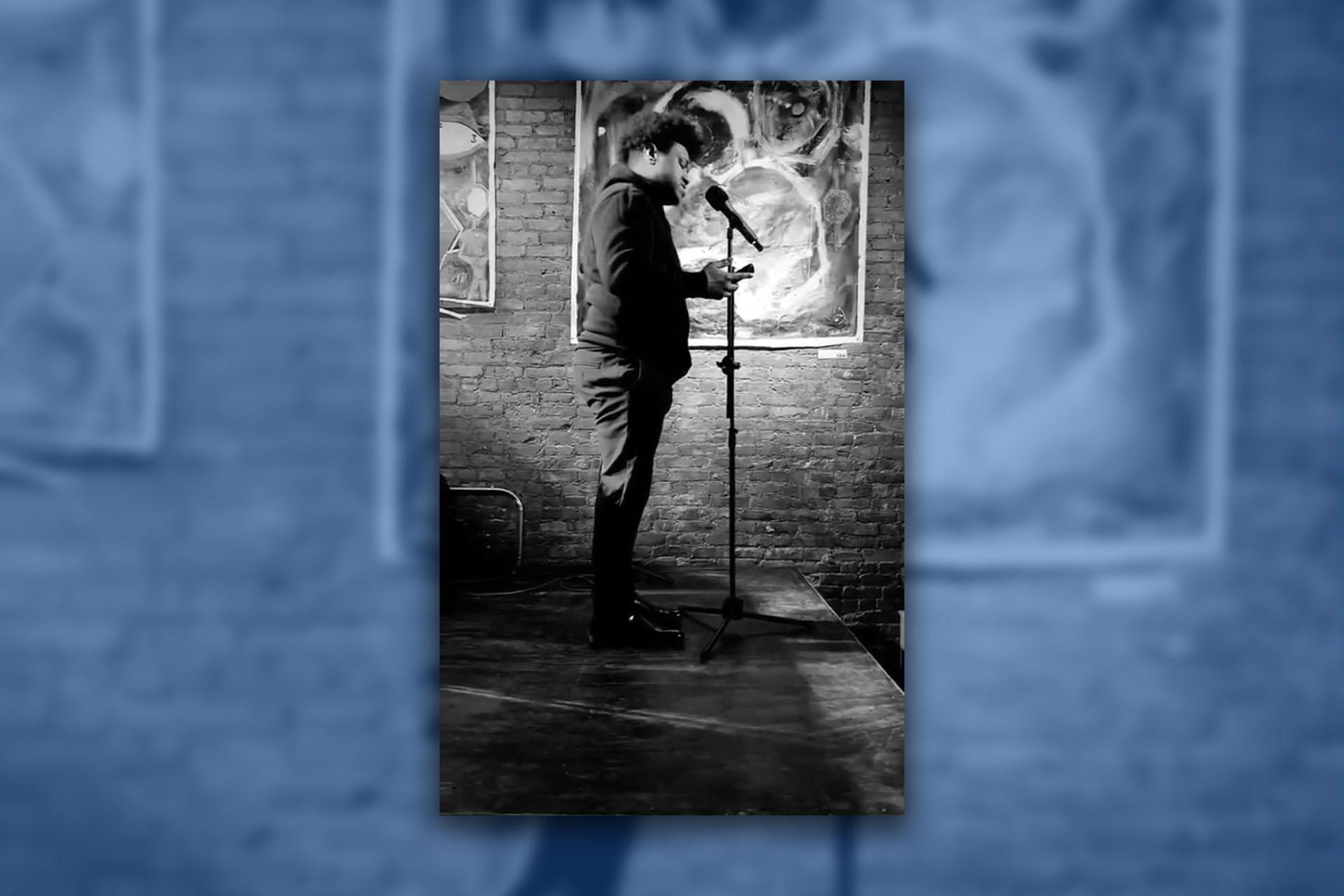The image captures a black and white photo of an African-American man standing on a stage, set against a blue wall with a design or artwork on it. The man, who has a small puffy afro, is wearing a dark-colored long-sleeve hoodie and dark jeans. He is standing at a microphone stand, with one hand possibly holding the microphone stand and his other hand down by his side or in his pocket. Behind him, there is an artwork and a large brick wall, with some visible pipes. The image suggests that he might be performing stand-up comedy or giving a speech.